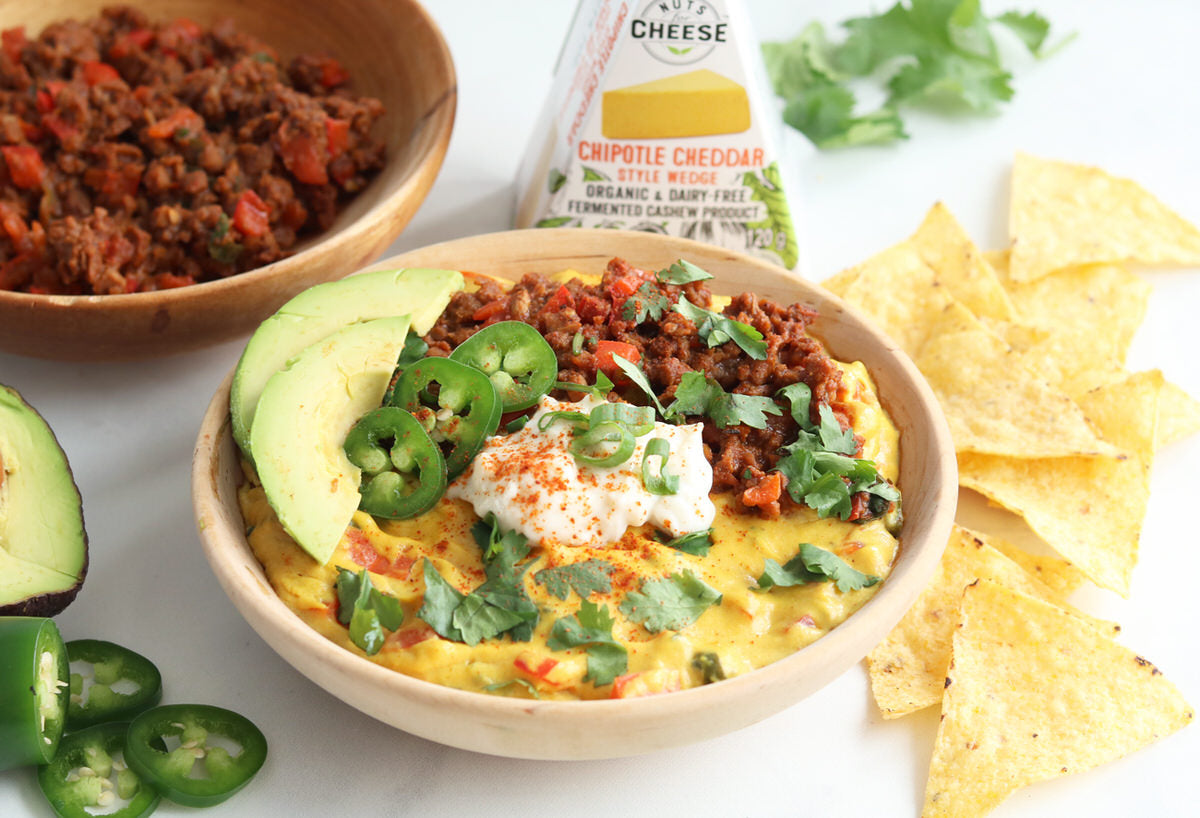The image showcases a professional photograph of a mouthwatering spread, featuring primarily two bowls of savory dishes set against a backdrop of a branded product packaging that reads "Nuts Cheese" with a visual of cheese shred. The focal packaging highlights "Chipotle Cheddar Style Wedge" in red text and "Organic and Dairy-Free Fermented Cashew Product" in black, with green accents.

In the upper left-hand corner, a brown wooden bowl contains a flavorful mix resembling chorizo or ground hamburger, enhanced by chopped onions, cilantro, and tomatoes. The central tan ceramic bowl is brimming with a hearty concoction that appears to be chili, complete with red peppers, slices of green jalapeno, part of an avocado, and finished with a dollop of white cream that might be sour cream, garnished with paprika and chopped scallions. Additionally, this bowl features layers of chorizo or fried hamburger, sliced avocados, a fried egg in the middle, scrambled eggs, and chopped cilantro. Other components scattered around include yellow tortilla chips in the lower left-hand corner.

Overall, the photograph beautifully captures the contrasting textures and vibrant colors of the ingredients, highlighting a delicious and visually appealing meal with elements of both authenticity and modern dietary preferences.